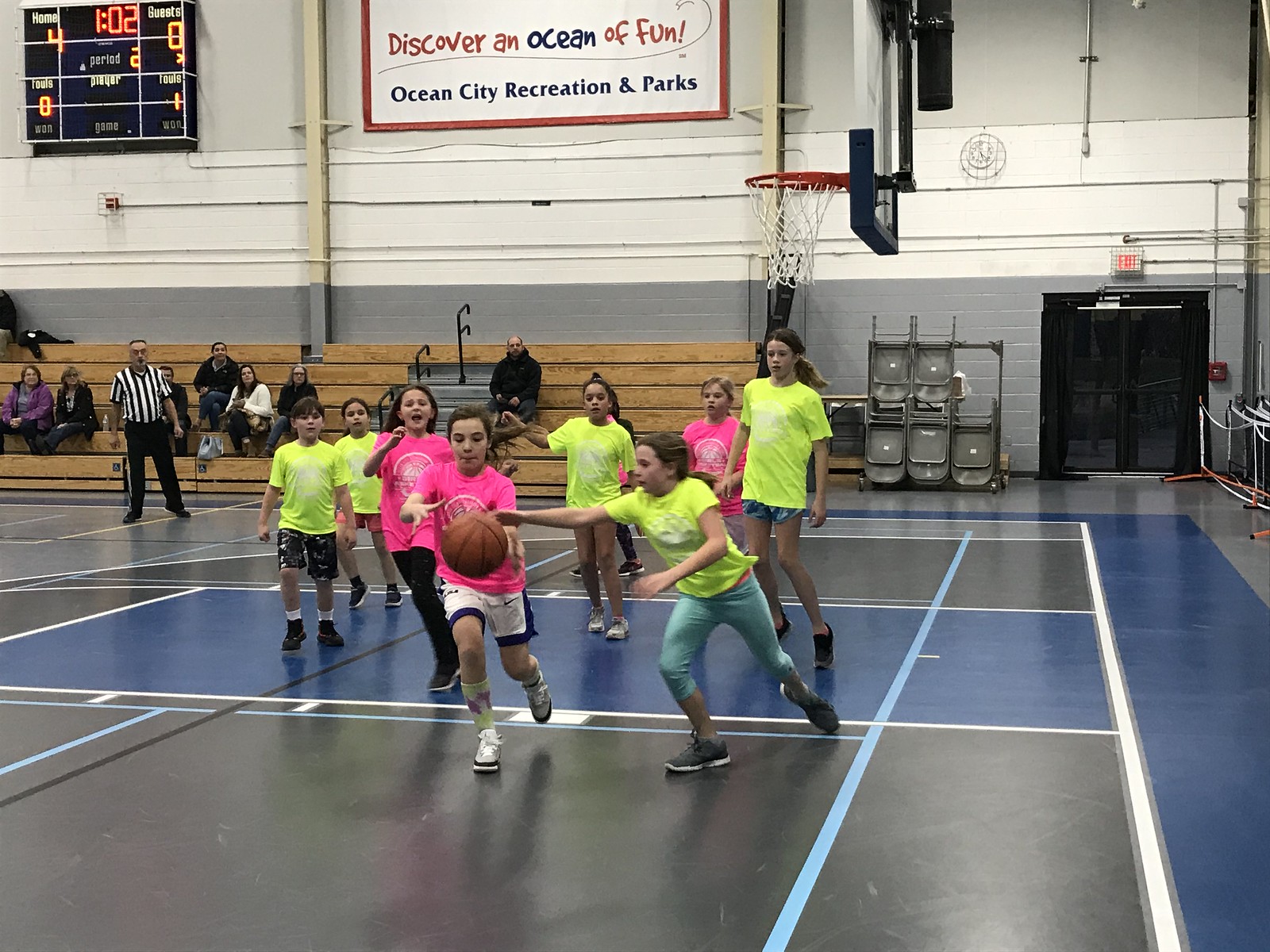An indoor game of basketball is captured in a color photograph featuring young children energetically competing on a black court with distinct blue, white, and dark black lines. Dominating the action in the foreground, a child in a light green shirt stretches towards a mid-air basketball, while a player in a light blue shirt and another in a pink shirt also reach out for the ball, intensifying the moment. Among the players, six wear light green shirts, and three sport light blue shirts. A referee, dressed in a traditional black and white striped uniform, stands watchfully in the upper left corner. Behind the lively game, wooden bleachers rise about five to six feet high, occupied by a few spectators. The gymnasium wall displays a sign that reads "Discover an Ocean of Fun, Ocean City Recreation and Parks." High above on the left, a digital scoreboard shows "Home 4, Guests 0," and a clock counting down from 1:02 during the second period. On the right side of the image, there's a doorway marked with a fire exit sign and chairs stacked together in a carriage.